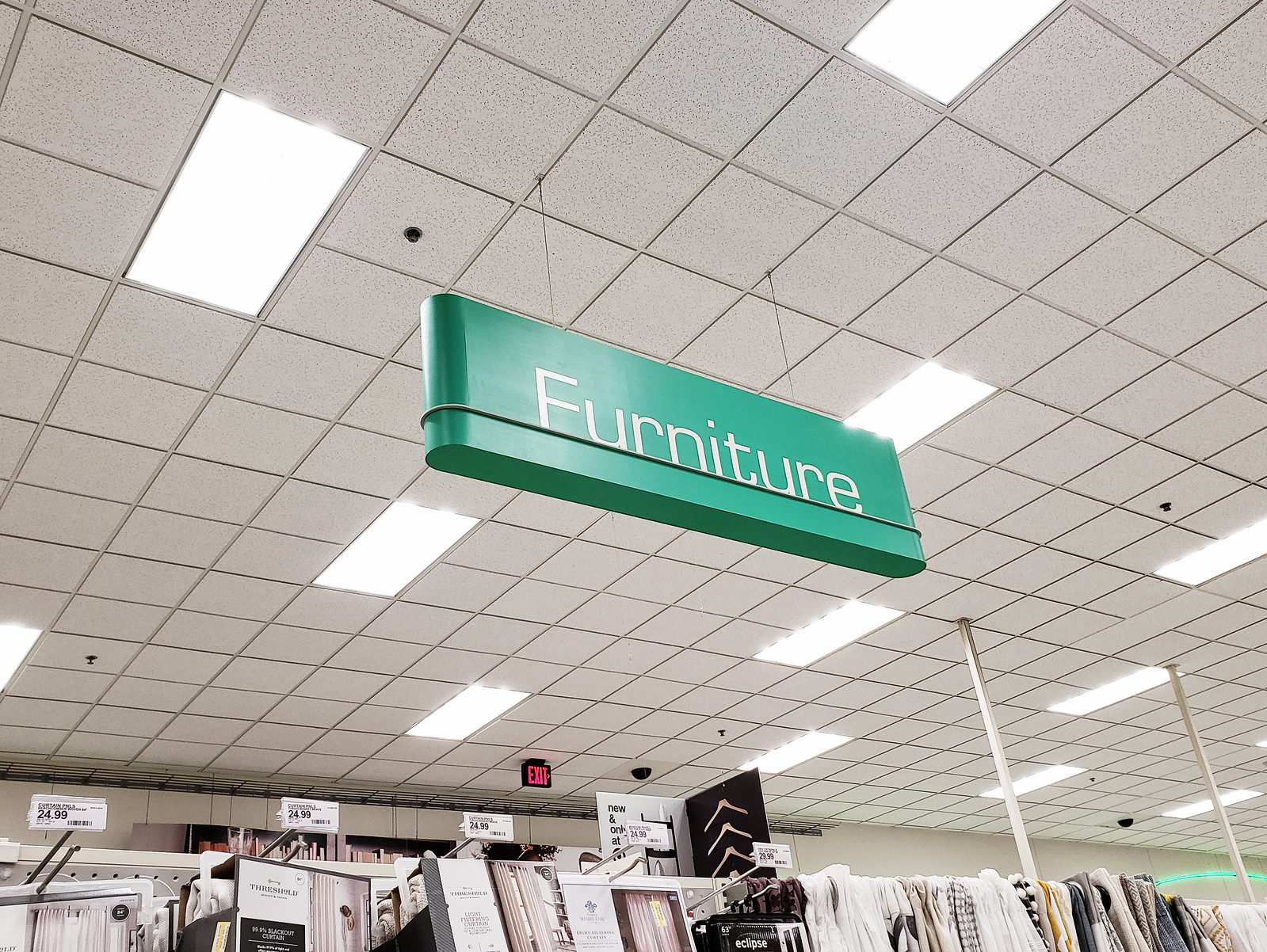This detailed and cleaned-up description of the image is as follows:

This is a color photograph taken indoors within a retail store. The perspective is angled upwards, revealing the ceiling composed of grey square tiles interspersed with rectangular white lights. A rectangular green sign hangs prominently from the ceiling, displaying the word "Furniture" in white lettering. 

At the lower part of the image, shelves or rails filled with either boxes or other items in black and white can be seen, although the contents are not clearly visible. White price tags are attached to the shelves, and a small, indistinct black and red sign hangs near the ceiling in the background. Towards the right-hand corner of the image, there appear to be additional rails, possibly holding clothing or fabric items. Above these rails, a small, illuminated green cord is visible, adding a touch of light to the scene.